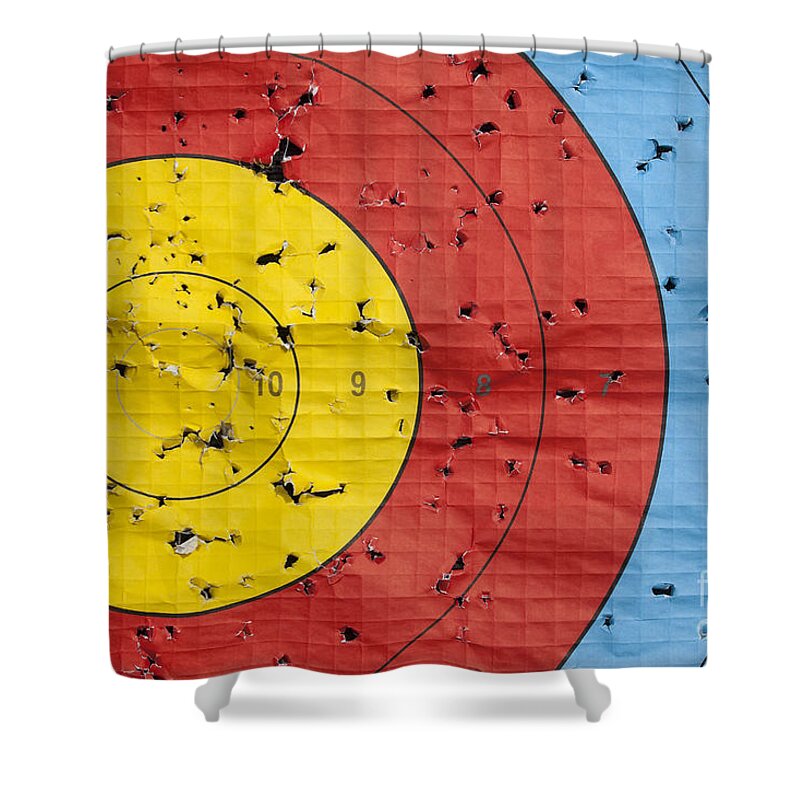This image features a shower curtain designed to resemble a dartboard or bullseye target, set against a white background. The shower curtain is suspended from a white curved pole at the top, held by several metal or black rings. The target pattern on the curtain is incomplete, truncated on the left, right, and top. The design consists of concentric circles with two sections of yellow in the center (marked with scores 10 and 9), followed by two red sections (marked with scores 8 and 7), and the outermost circle in blue. Scattered across the curtain are numerous holes, creating the illusion that it has been repeatedly hit by darts. At the very bottom of the image, below the curtain, two white legs of a bathtub are visible.